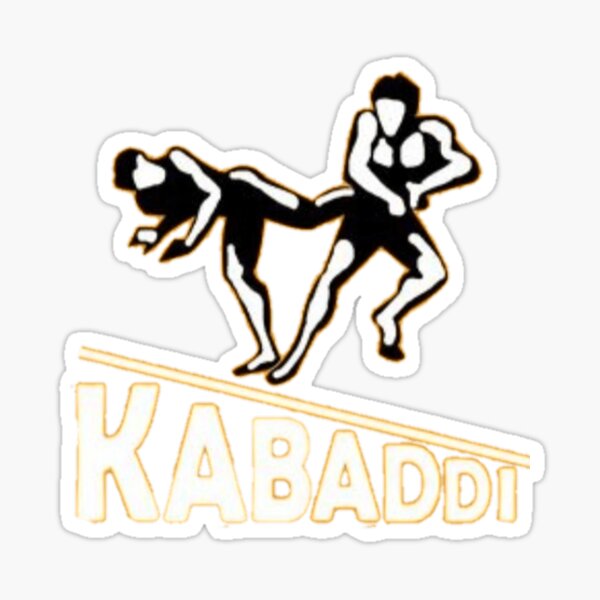The image features a square decal or sticker with a light gray background, depicting two black silhouettes of human figures engaged in a combat-like pose, similar to kickboxing. The figure on the left is balanced on one leg, executing a kick towards the figure on the right, who appears to be attempting to grab the kicker's leg. Both figures are dressed in black from the chest down to their mid-thighs, and they are wearing gloves. The combat scene is set above a bold, white label with gold bars and the word "KABADDI" in big, capital letters, outlined in orange. The label has two red lines representing the ground beneath the fighters.